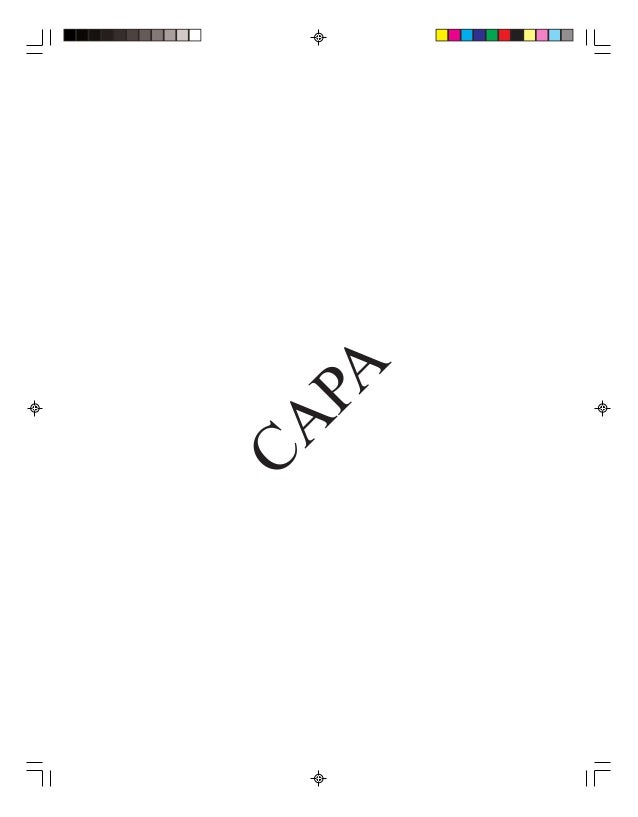The image appears to be a printer test page, set against a completely white background. At the top left, there is a series of boxes displaying a grayscale gradient, transitioning from dark black on the left to bright white on the right. In the top right corner, there is a collection of color boxes featuring various colors: yellow, red, blue, purple, green, orange, light pink, light blue, and gray. Positioned diagonally across the center of the image, the word "CAPA" is prominently displayed in black, all-caps Times New Roman font, angled at 45 degrees from the bottom left to the top right. Surrounding the edges, there are multiple circular targets, each set at the top, bottom, left, and right sides. Additionally, each corner of the image features a 90-degree angle mark, accompanied by a line extending downward and to the left.